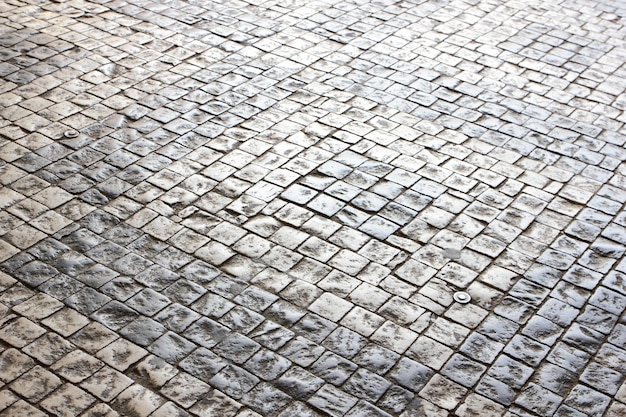This color photograph, likely taken outdoors during the daytime, showcases a stone street or walkway reminiscent of those found in downtown Brooklyn around Williamsburg and Dumbo. The surface is composed of small, square tiles arranged in a distinct pattern: alternating light beige and dark gray squares, with darker gray squares in the center of each pattern. The stones are visibly aged and weathered, featuring black dirt in the crevices and a bumpy texture suffused with wear. Interspersed among the stones are small round discs made of plastic and metal, possibly nails or casings, which can be seen on both the right and left sides of the image. The presence of daylight is evident, highlighting the intricate details and the rustic charm of this urban pathway.